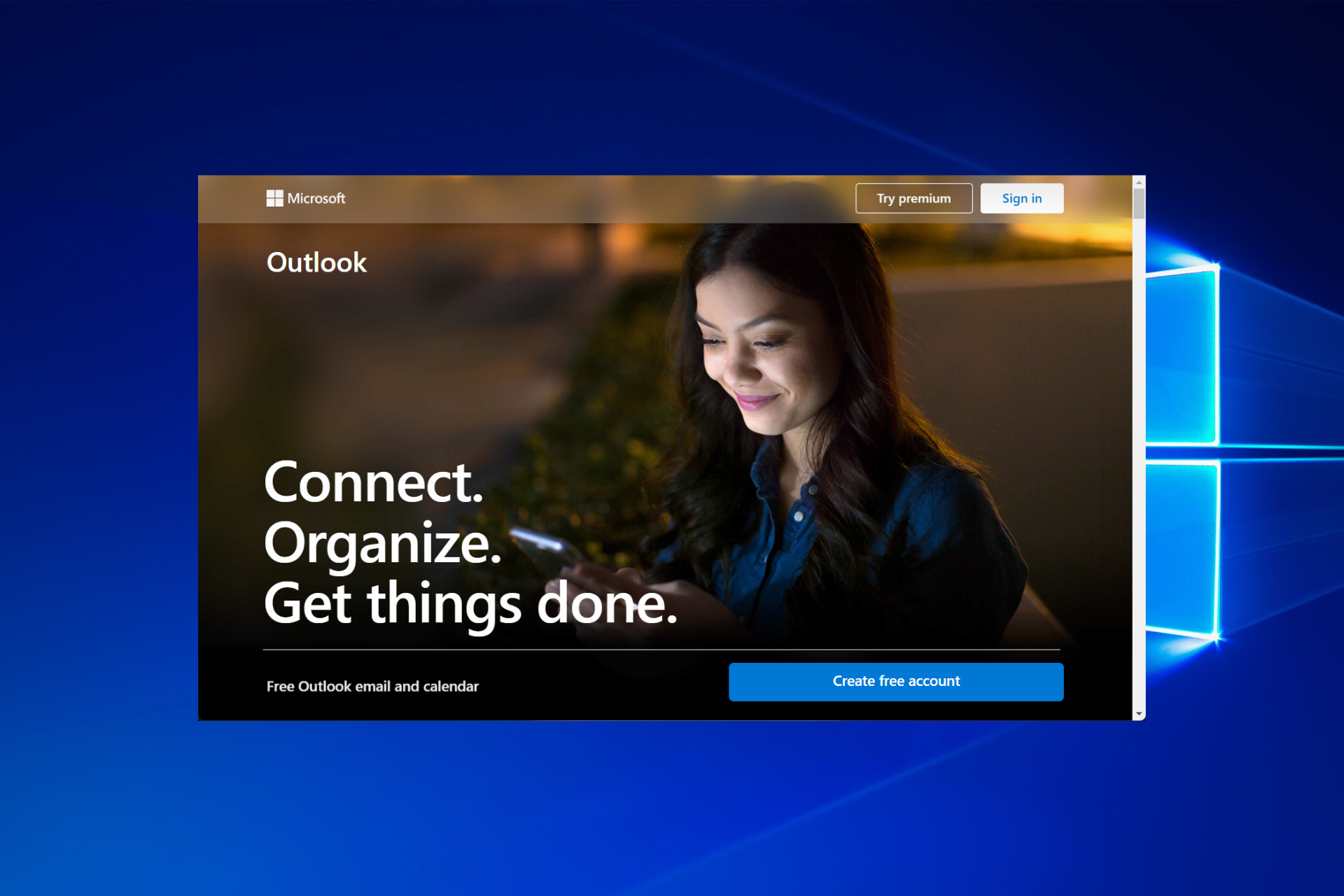This is a detailed screenshot of a Windows browser showcasing a promotional page for Microsoft Outlook. At the forefront, there is a high-quality image of a woman with long, dark brown, curly hair, dressed in a blue blouse. She is smiling and looking down at her phone, exuding a sense of focus and satisfaction.

To the left of the woman, in large white text, are the words "Connect, Organize, Get Things Done," emphasizing the core values of the Outlook application. At the top left corner, the Microsoft logo and the word "Microsoft" are displayed in a smaller font, forming part of a header that is overlaid across the top of the image. To the right side of this header, there are two prominent buttons: one labeled "Try Premium" and the other labeled "Sign In."

Beneath the Microsoft logo within the image, the word "Outlook" is prominently featured, creating a distinct separation from the top header. At the very bottom of the screenshot, a separate footer is visible. This footer contains the text “Free Outlook Email and Calendar” on the left and a long blue rectangular button that says "Create Free Account" on the right.

The woman in the image occupies the central part of the screen, surrounded by a blue background featuring glowing squares to the right, with light emanating through the squares also from the right. This design choice adds a high-tech and modern aesthetic to the overall composition.